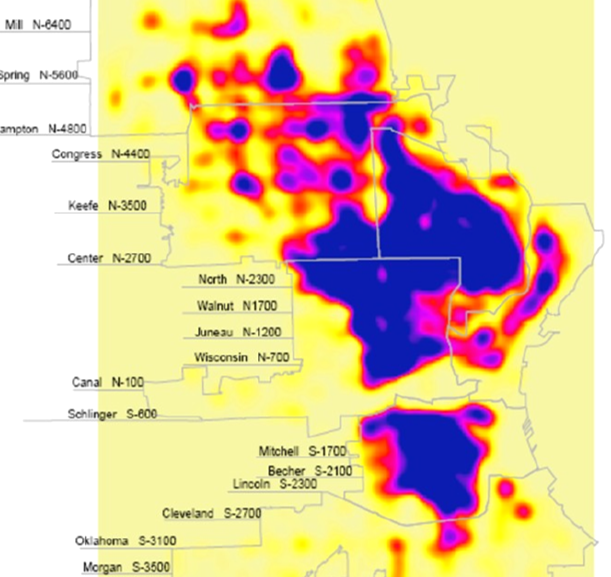The image is a thermal map overlaid on a region divided into various territories marked by numerous black-text labels and numbers, resembling counties or districts. Primary background color is yellow, transitioning to darker tones with reds, purples, and blues indicating varying thermal intensities -- with dark blues representing the most extreme temperatures. Amidst this, there's a spectrum of colors illustrating the thermal imaging, extending from the top-left to the bottom-right of the map. Key street names and numerical designations, such as Spring N5600, Hampton N4800, and Lincoln S2300, are spread across the map, with lines intertwining through and around these labels to delineate specific areas. Additional text markings frame the image, originating from outside and moving into the map, enhancing the detailed segmentation of the represented regions.